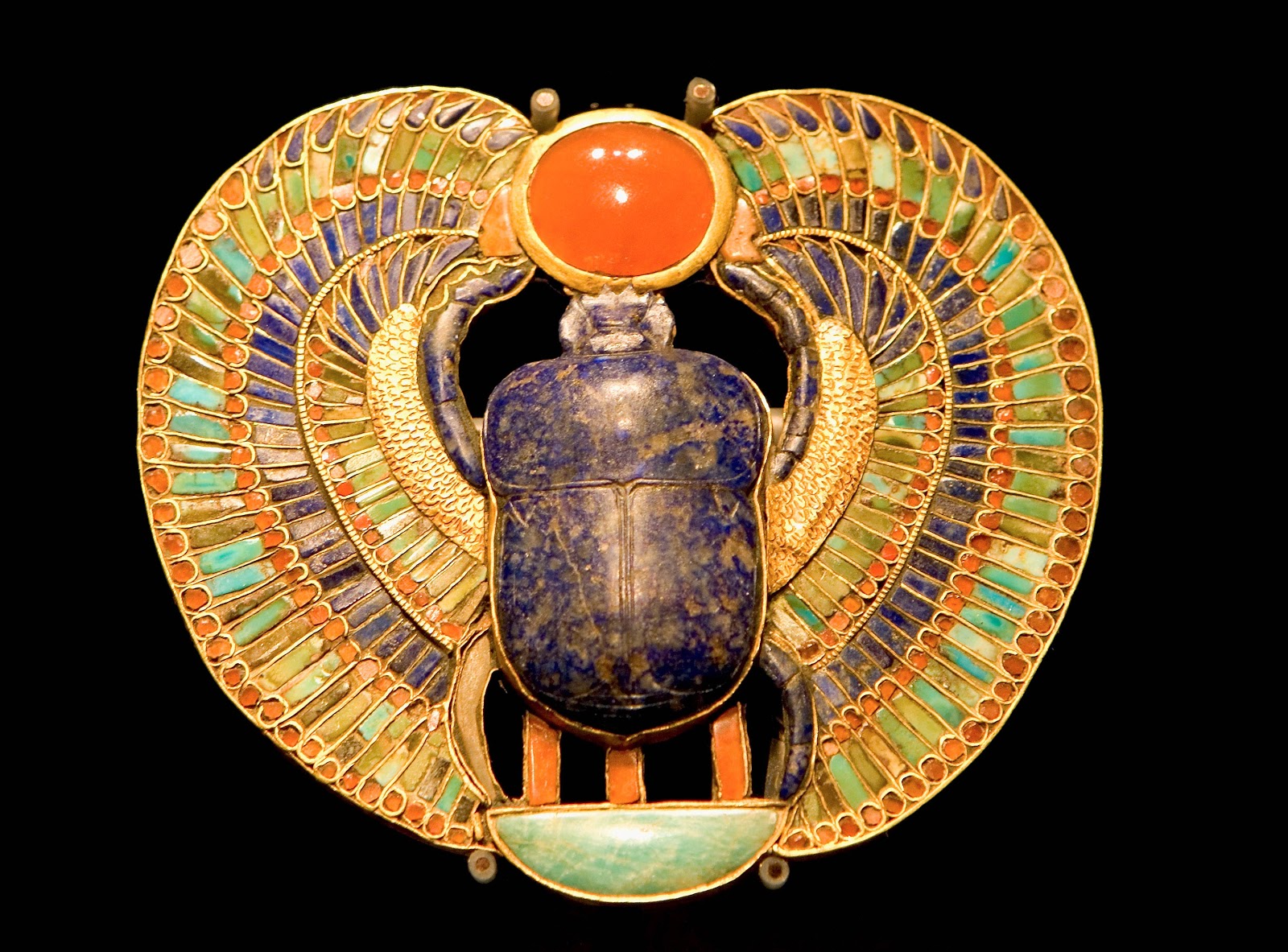The image showcases a highly detailed and ornate piece of jewelry resembling an ancient artifact. At the center lies a black beetle with a brownish-black hard shell, topped by a head that is a mix of off-white and black, encircled in gold. The beetle's head features prominent antennas and is surmounted by an orange circle with gold trim, as wide as the beetle itself. The beetle's elongated back shows intricate sections: the top section is rectangular, while two dark blue segments with hints of rust run underneath. Gold-framed wings stretch out from the central orange circle, each adorned in elaborate patterns of blue, red, purple, green, and orange hues.

From the beetle's back, extending downward, are three slender orange rectangles meeting at a blue, gold-trimmed half-moon at the creature's hind legs. These back legs point downward and are also blue. The entire artifact rests against a black background, bringing out the vivid colors and meticulous craftsmanship of the piece.